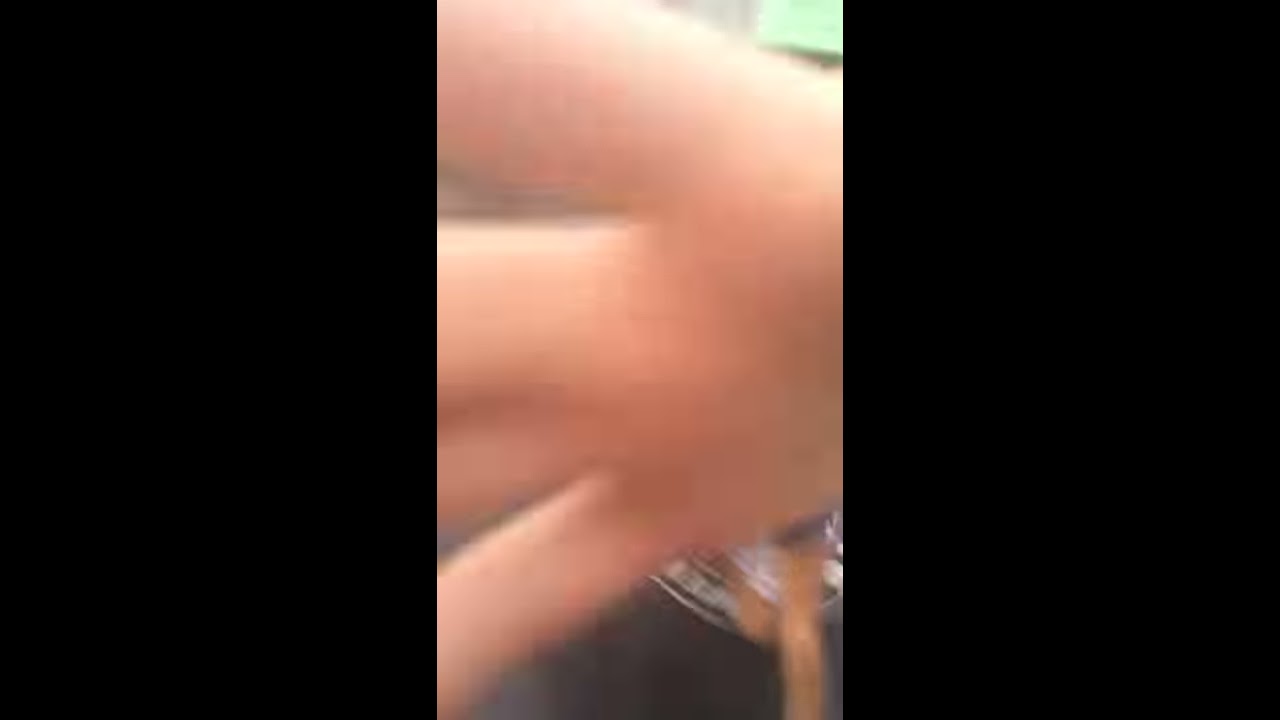The image is a highly blurred, close-up photograph primarily dominated by a hand attempting to block the lens, creating a central focus on the palm and a part of the fingers. The left and right thirds of the image are entirely black, providing a stark contrast to the blurred center. Visible details include the inner side of the hand, with the area extending from just below the first knuckle to the palm, occupying about 80% of the frame. The bottom portion suggests a dark-colored floor, possibly black or dark brown, with the faint outline of bare feet clad in dark pants. In the upper-right corner, a light green hue hints at an object like a fish tank or perhaps a view through a window, though it remains indistinct. The image behind the hand is indistinguishable, with mentions of a possible metal object and something hanging down, adding to the overall ambiguity.